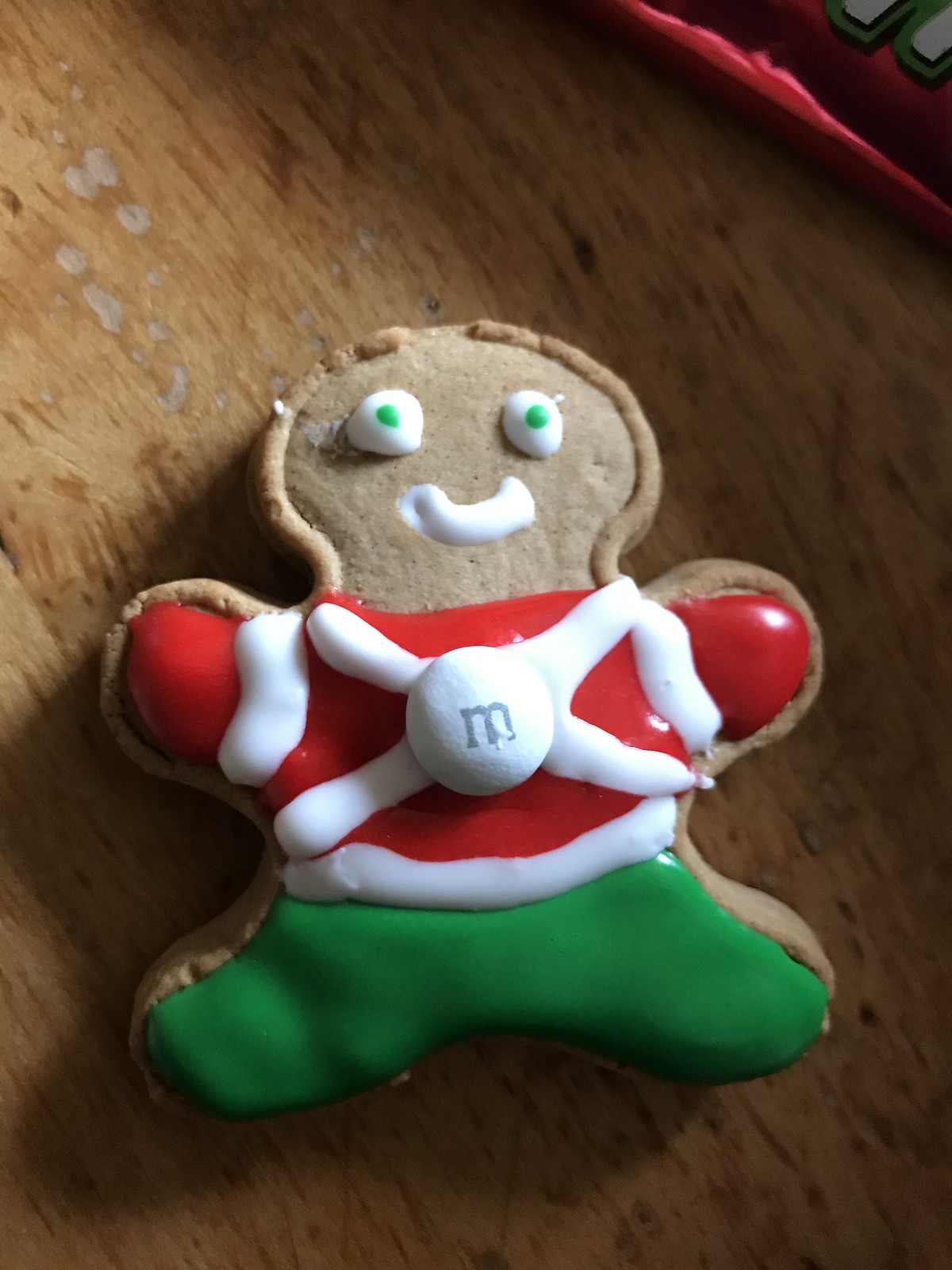The image showcases an old, weathered wooden background, marked with nicks and scratches, possibly a brown wooden plate. Centered on this rustic backdrop is a gingerbread cookie, characterized by its light brown, bear-like head. The cookie's eyes are green with white icing details, and it has a white smiley mouth. The gingerbread figure wears a red shirt adorned with a white X pattern made from icing, featuring a white M&M candy in the center of the X. The pants of the figure are a lighter green color. A subtle brownish trim around the head gives the appearance of hair, adding to the festive, holiday-themed design with its classic Christmas colors of red, green, and white.